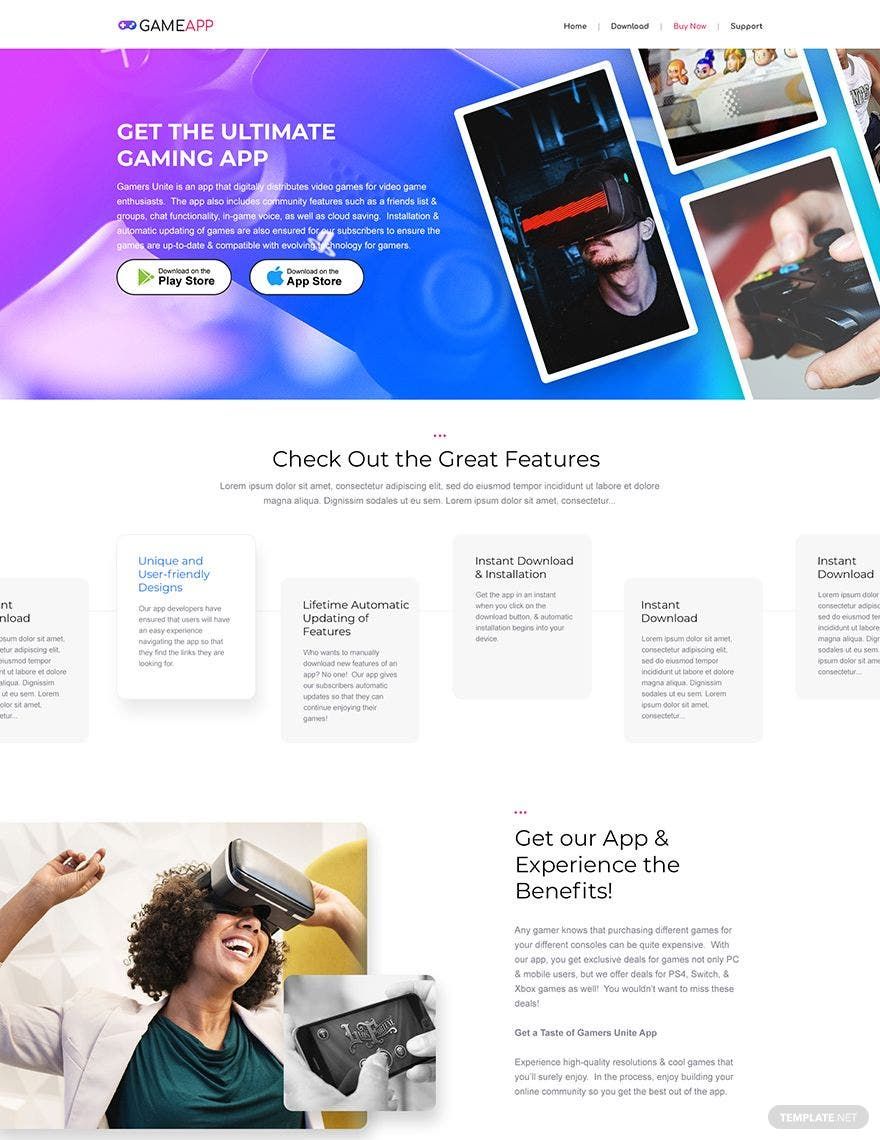The image is an advertising page for the 'Gamers Unite' app, designed for video game enthusiasts. In the top left corner, a purple video game controller icon accompanies the title "Game App." Adjacent to it is a menu offering options like Home, Download, Buy Now, and Support. Dominating the upper central section, text reads "Get the Ultimate Gaming App," promoting 'Gamers Unite'—an app known for digitally distributing video games and featuring community-oriented functionalities such as a friends list, groups, in-game voice, and cloud saving. The app ensures automatic updating and easy installation of games to keep them up-to-date and compatible with emerging technologies. Two prominent download buttons for the Play Store and the App Store encourage users to get the app.

Moving further down, the bottom two-thirds of the page highlight various features under the header "Check Out the Great Features," though the following detailed descriptions are obscured by placeholder text (Alorum, Ipsum, Dolar, Cimet). Illustrative boxes hint at different functionalities, but their accompanying text is too small to decipher. Visual elements enrich the advertisement: an African American woman wearing a VR headset is positioned in the bottom left, her arm raised in excitement, and a smaller inset image shows someone playing a mobile game on a phone. Additionally, small scattered images illustrate people using a gaming controller or a VR headset, enhancing the interactive impression of the app. The blue border at the top and additional red background elements with gaming controllers and PlayStation imagery add vibrant visual depth to the page.